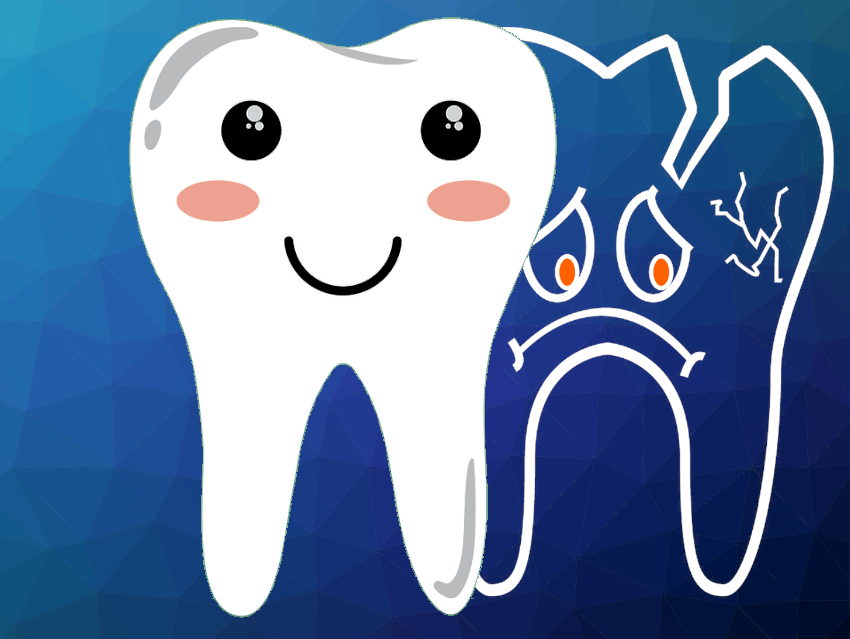The image features two cartoonish molar teeth against a gradient blue background composed of geometric triangular shapes that create a 3D textured look. On the left side is a happy, healthy white tooth adorned with black beady eyes, rosy cheeks, and a broad smile shaped like a U. This tooth is simplistic in an anime art style, appearing bright and smooth with a hint of gray shading to imply shine and detail. In contrast, on the right side of the image is a sad, transparent tooth with orange eyes and a sorrowful expression. This tooth shows visible signs of damage, including a significant crack at the top and another along the top right edge, contributing to its unhappy demeanor. The detailed artwork and clear lighting highlight the contrasting conditions of the two teeth, making the overall image vibrant and easy to comprehend.